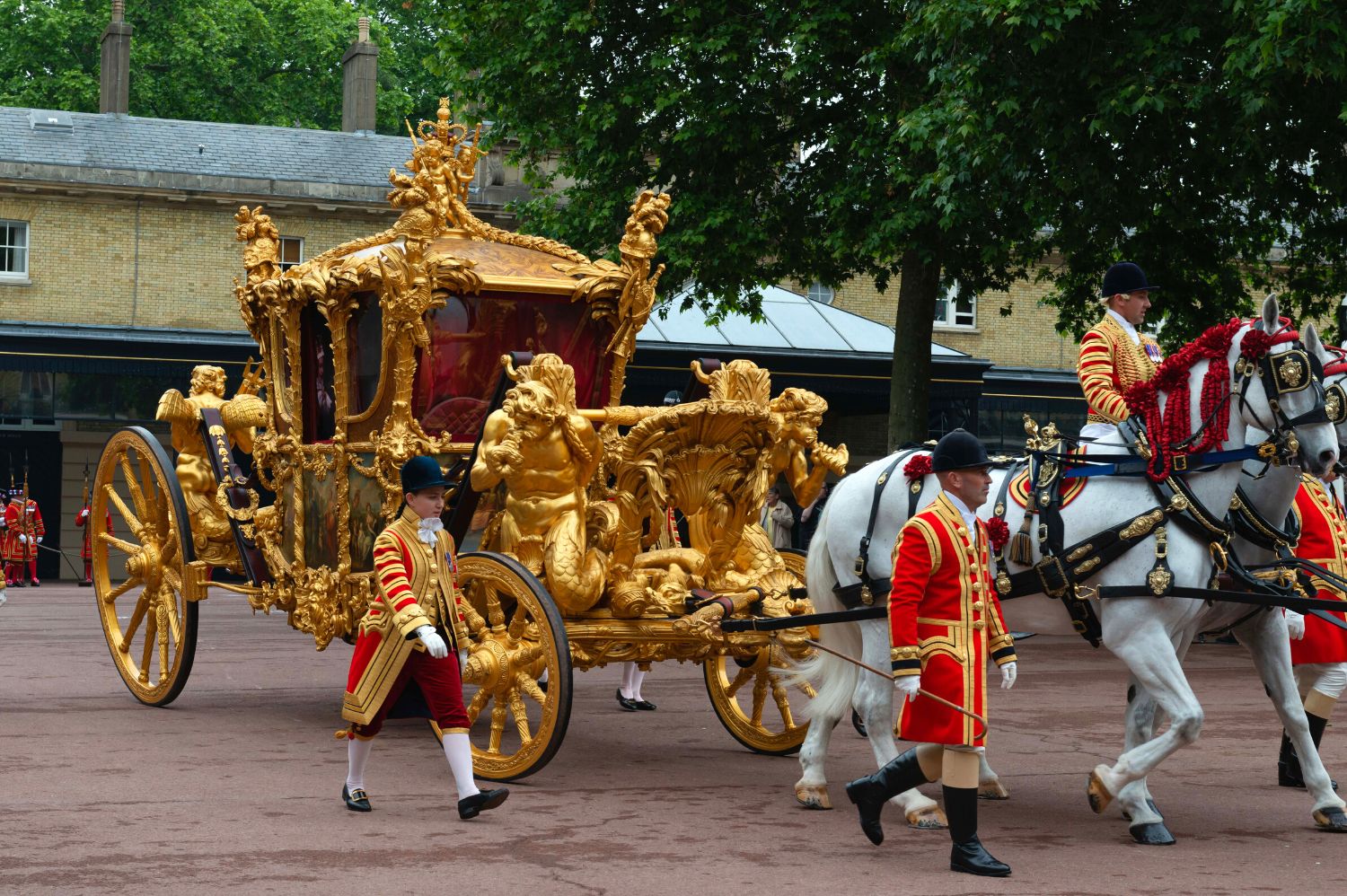In this richly detailed image, a highly ornate gold carriage reminiscent of a royal coach or Cinderella's carriage takes center stage, occupying two-thirds of the frame as it prepares to depart from a stable area. The majestic vehicle is adorned with intricate statuary, including a naked angel or herald blowing a horn, announcing the presence of its esteemed occupant. Four golden wheels with black rubber spokes support the resplendent carriage, which is surrounded by trees and a house in the background.

Two beautifully decked-out white horses pull the carriage, their manes embellished with red adornments. One of the horses is being ridden by a jockey, while several people in dazzling red and gold uniforms accompany the procession. Additional figures clad in orange and yellow outfits are present, adding to the grandeur of the scene. The carriage is accompanied by mermaid-like statues with gold fins, further enhancing its extravagant appearance. The solemnity and beauty of the scene, possibly part of a parade or procession, captures the viewer's attention, making it a captivating image to behold.